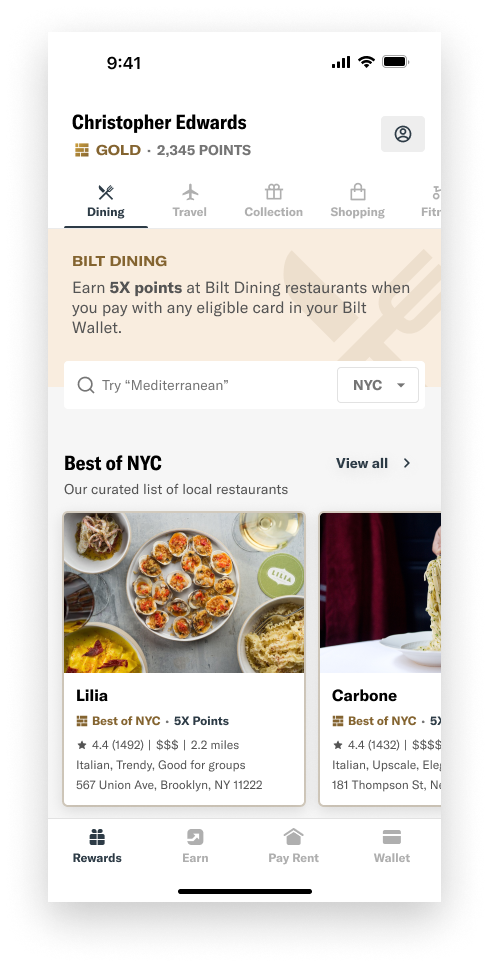A detailed screenshot showcase of a mobile application interface:

At the top of the screen, there is a white header displaying the current time "9:41" in black font, slightly indented on the top left. On the top right, three black icons are arranged in sequence.

Beneath the header, towards the left side, bold black text reads "Christopher Edwards." Below the name, there is an icon of stacked golden bars featuring a shiny tinge. To the right of this icon, the text "GOLD" is written in all caps in gold color. Adjacent to this, a medium gray dot separates the text from "2345 points" written in medium gray color. Aligned to the right of these elements, a light gray square with rounded corners hosts a black profile picture icon.

Below this section, several tabs are laid out. The first tab on the left features a black icon of crossed knife and fork, with the bold black text "DINING" under it, followed by a thin black underline. The subsequent tabs follow a similar design in medium gray without an underline: an airplane icon for "TRAVEL," a gift icon for "COLLECTION," a shopping bag icon for "SHOPPING," and an additional cut-off tab whose content is not fully visible.

Underneath these tabs, a beige header contains gold text on the top left reading "BUILT DINING" in all caps. Below this header, gray text declares: "EARN FIVE TIMES POINTS AT BUILT DINING RESTAURANTS WHEN YOU PAY WITH ANY ELIGIBLE CARD IN YOUR BUILT WALLET." The phrase "Five times points" is emphasized in bold, with "five times" represented by the numeral "5X." The rest of the page content extends below this section.